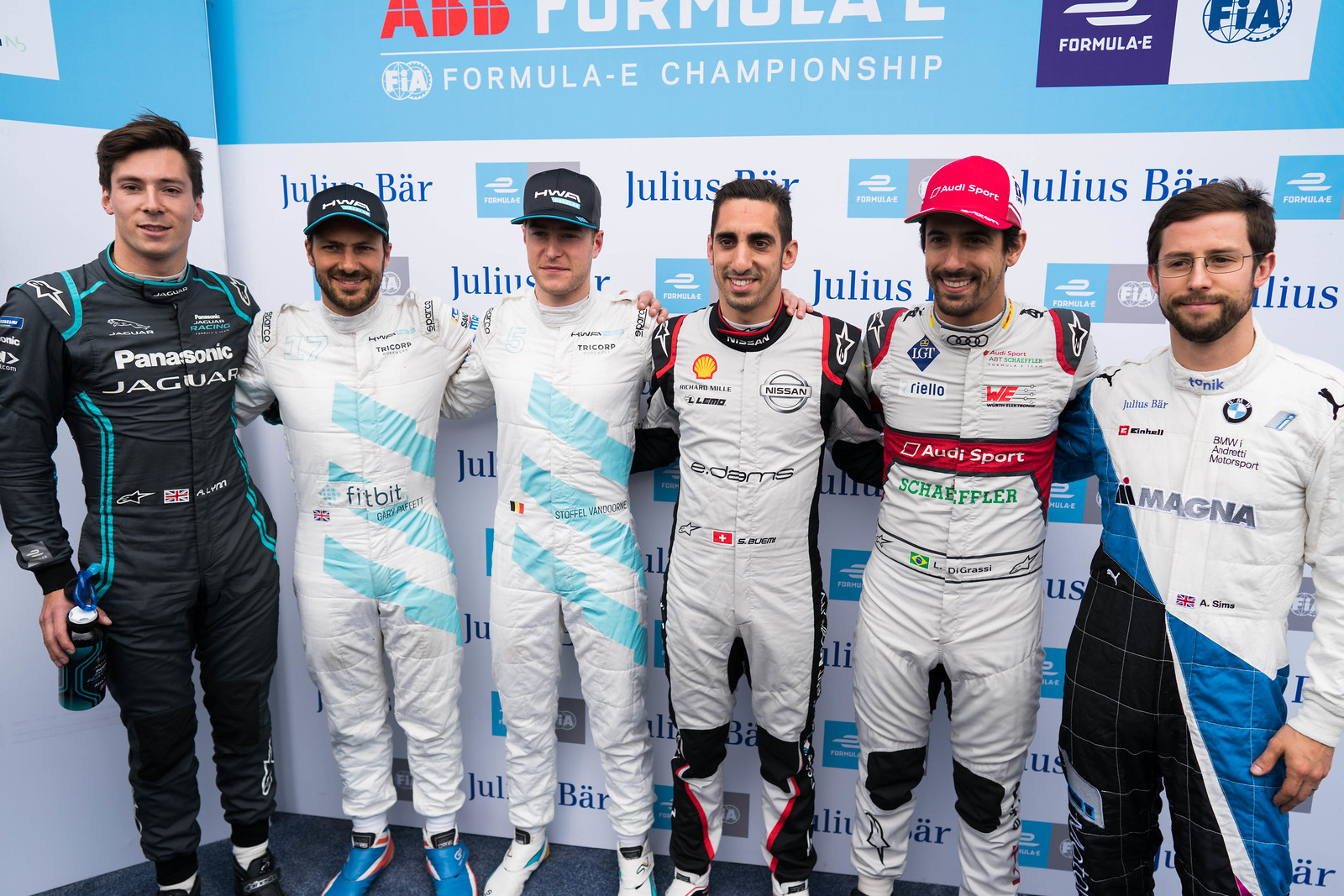The image showcases a group of six Formula E Championship race car drivers standing in front of a vivid blue and white display adorned with the event's branding and sponsor logos, including "Julius Baer" and "ADD Performance." The driver on the far left sports a mostly black racing suit with cyan stripes, branded with "Panasonic" and "Jaguar," and holds a black and green drink bottle. The next two drivers, both wearing white uniforms with light blue and black accents, feature "Fitbit" and "TriCorp" sponsorships along with names "Stoffel Vandoorne" and "Gary Paffett." The fourth driver dons a black, red, and white suit with the name "Adams" on it and has short black hair. Standing next to him is a racer in an Audi Sport red hat and a black, white, and red uniform. The last driver wears a white, black, and blue suit. Three of the drivers wear black caps, while one wears a red cap. They stand closely together with arms around each other’s shoulders, exuding camaraderie and smiles for the camera.